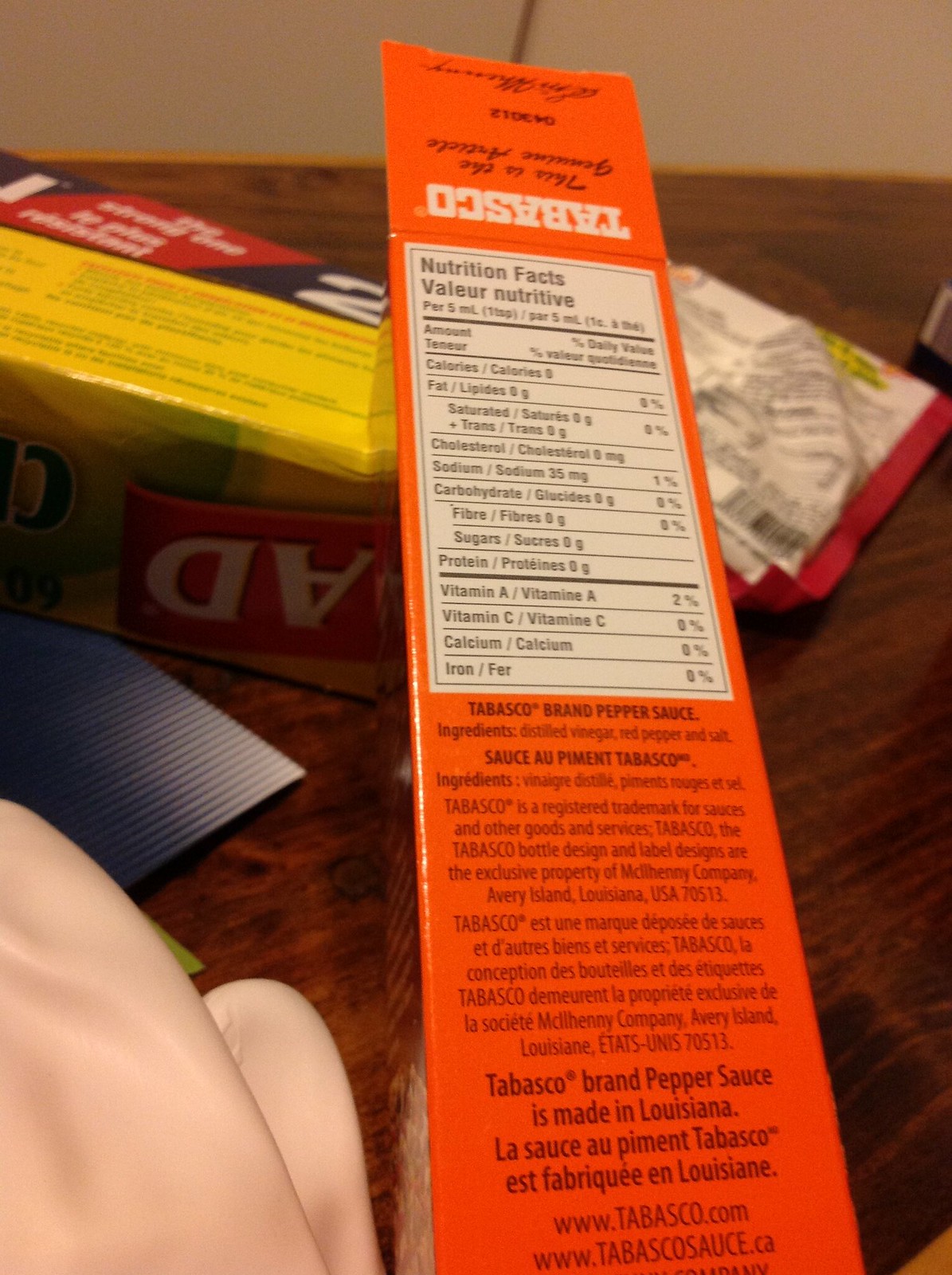This detailed photograph captures a chocolate brown hardwood table laden with various items, with the focus on an orange box of Tabasco pepper sauce, prominently displaying its Nutrition Facts label. The label presents detailed nutritional information per 5 milliliters, highlighting 0% fat, cholesterol, fiber, and carbohydrates, with 1% sodium and 2% vitamin A, alongside ingredients such as distilled vinegar, red pepper, and salt. This box also indicates that Tabasco is a registered trademark, made in Louisiana, with an accompanying French translation and the website www.tabasco.com.

To the right, a yellow box of Glad Cling Wrap lies on its side, partially overlaid by the Tabasco box. The Glad box features red and white text, with portions of its green and black labels visible. Nestled in the upper right-hand corner is a square, small packaging, possibly a packet of taco seasoning, alongside a white bag trimmed in red.

In the bottom left, a piece of pink material, likely clothing, peeks out, with a shiny metallic square positioned above it. To the top left, another blue package with red and white labeling can be glimpsed, while the backdrop includes a hint of a white wall. The ensemble of items on the rich wooden table creates a richly textured and detailed composition, dominated by the vivid orange Tabasco box.